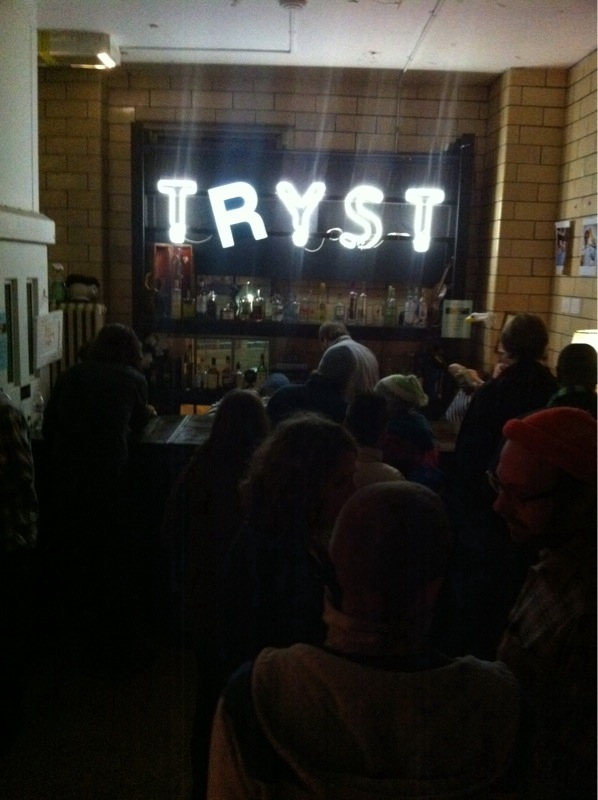The image depicts a bustling bar interior with low light and rustic brick walls, creating a cozy yet vibrant atmosphere. The room is crowded with patrons who are predominantly gathered on the right side, while the left side remains intriguingly open. In the center of this scene is a wooden bar counter, behind which stands a solitary bartender. He is focused intently on the shelves below him, stocked with an assortment of liquor bottles. Above these shelves, a striking neon sign illuminates the area with stylized white letters spelling out "Tryst," though the 'R' in the sign is distinctly different in style, set apart by having no gaps unlike the other letters. The overall setting exudes a mix of warmth and excitement, characteristic of a lively night out.